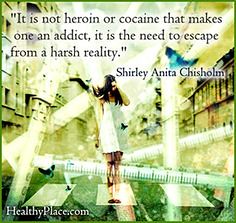The image is a small, square digital card from healthyplace.com, featuring a woman in a white dress with shoulder-length dark brown hair. The woman, who is standing on what appears to be a small platform, faces slightly to the left with her right arm extended, and her left arm in front of her face. The white dress depicts a butterfly, adding a touch of delicate detail.

In the background, there is a chaotic, colorful, and somewhat blurry mix of different elements including large medical syringes, faded buildings, and what appears to be a leaning tower on the left. The overall setting behind the woman is indistinct and dreamlike, emphasizing a sense of confusion and escape.

Overlaying the image at the top is a quote in black text: "It is not heroin or cocaine that makes one an addict, it is the need to escape from a harsh reality." The quote is attributed to Shirley Anita Chisholm, with her name placed underneath in smaller text. A small blue symbol appears near her name, possibly an arrow. This evocative image visually underscores the quote's profound message about addiction and escape.